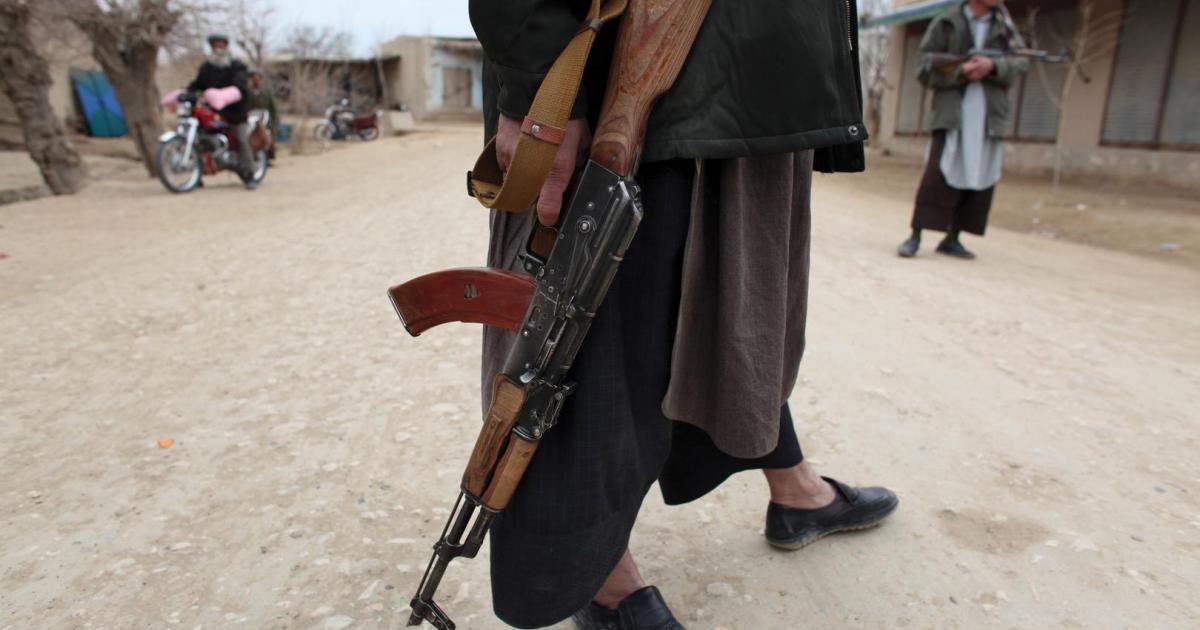In a rural Middle Eastern or Muslim country village, the image depicts a dirt street lined with small old houses and a tree in the background. In the foreground, the lower half of a man can be seen, wearing traditional Islamic garb: a dark-colored "skirt" or long tunic ending above his ankles, and a jacket. His feet are shod in black shoes without socks. He firmly grips an AK-47 in his right hand, finger on the trigger, the rifle featuring a long curved clip, wooden accents, a wooden stock, and a brown strap. To his right, another similarly dressed man in a gray jacket and blue "bermice" is also holding an AK-47. On the left side, a white-bearded man on a small motorcycle approaches, wearing a hat and conspicuously sporting pink kitchen gloves while gripping the handlebars. Another unoccupied motorcycle is visible behind him. The streets and surroundings highlight a rustic scene in a rural town.